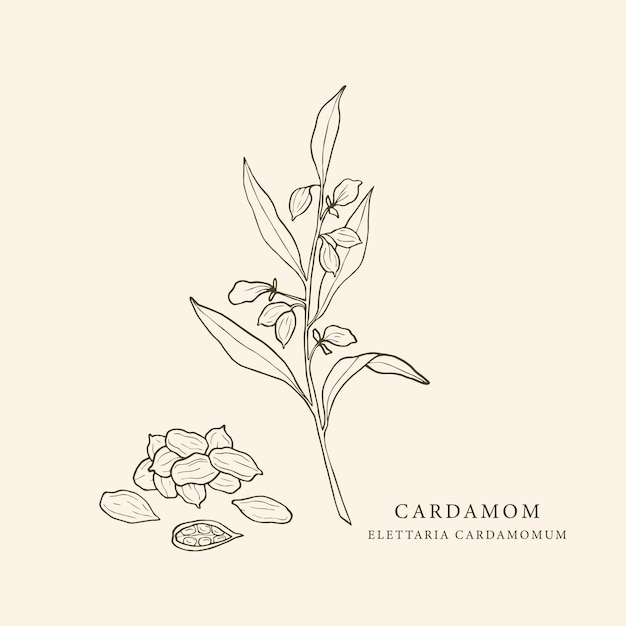This is a detailed, line ink drawing of a cardamom plant, likely from an herbal encyclopedia or scientific textbook, set against a beige background. The central focus is on a tall, slender diagram of the plant's structure, which showcases its elongated, graceful leaves and floral buds. The botanical illustration is meticulously labeled with the common name "Cardamom" and the Latin name "Elettaria cardamomum" on the lower right. To the left, there is a depiction of mature cardamom pods, some of which are shown in a pile. One pod is cross-sectioned to reveal the numerous tiny seeds within, which are harvested for their aromatic, medicinal, and culinary properties. The entire image is rendered in minimalistic black ink, emphasizing the plant's detailed anatomy without the use of color, enhancing its scientific clarity.